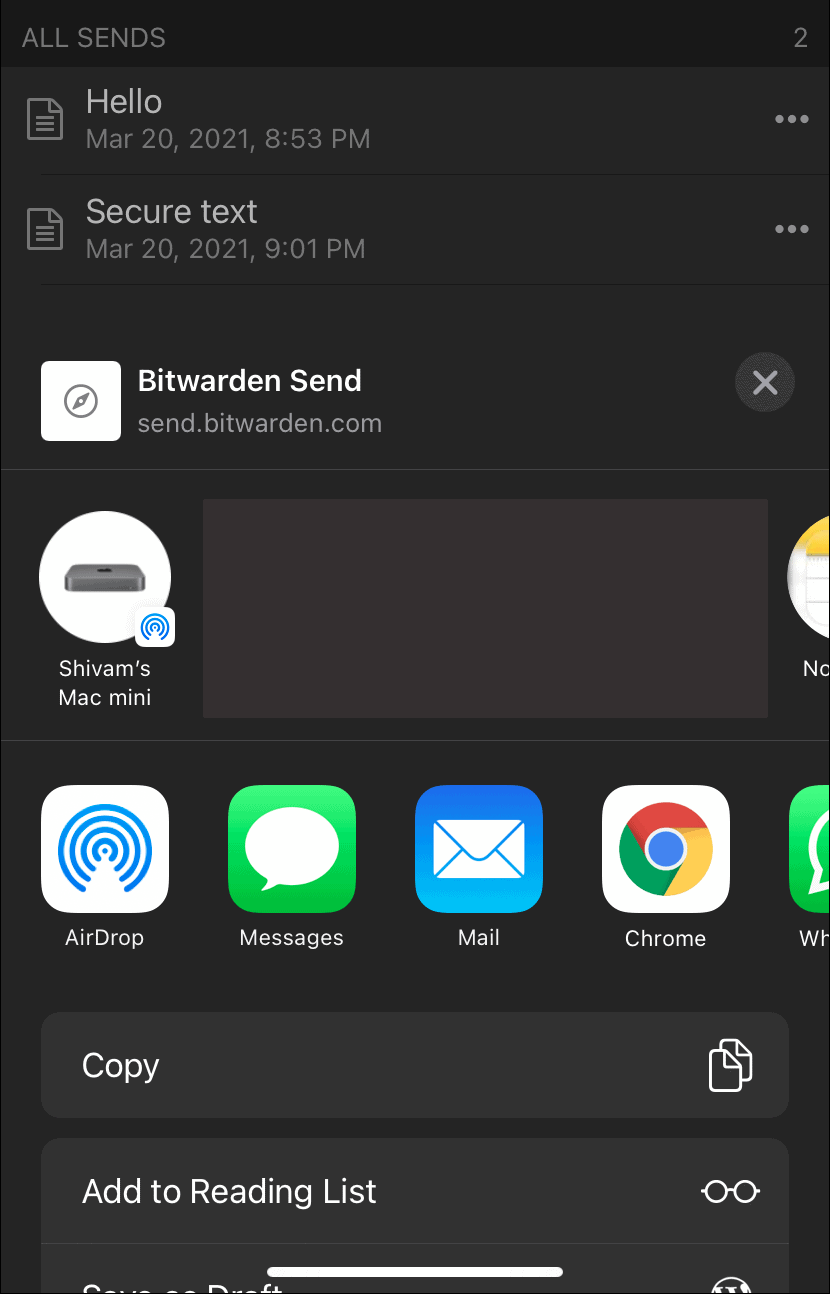The image displays a digital document marked with various timestamps and messages. The first timestamp reads "March 20th, 2021, 8:03 p.m." followed by the text "Document says: hello." Another timestamp on "March 20th, 2021, 9:01 p.m." indicates "Document says: secure text." The background is predominantly gray with a sequence of circular shapes; one is gray, and another is white. Further, there are multiple icons and text elements arranged in a grid-like pattern. 

A gray square icon labeled "Airdrop" is visible, followed by a green square labeled "Messages." The "Mail" icon is also present, labeled on a white square. The "Chrome" icon is displayed with its recognizable colors: red, yellow, green, and blue. Instructions to "Copy this way" lead to a reading list button, situated above a white bar at the bottom of the image. The composition features various types of text arranged in three rows, each differing in style, and numbering five visually distinct elements in total.